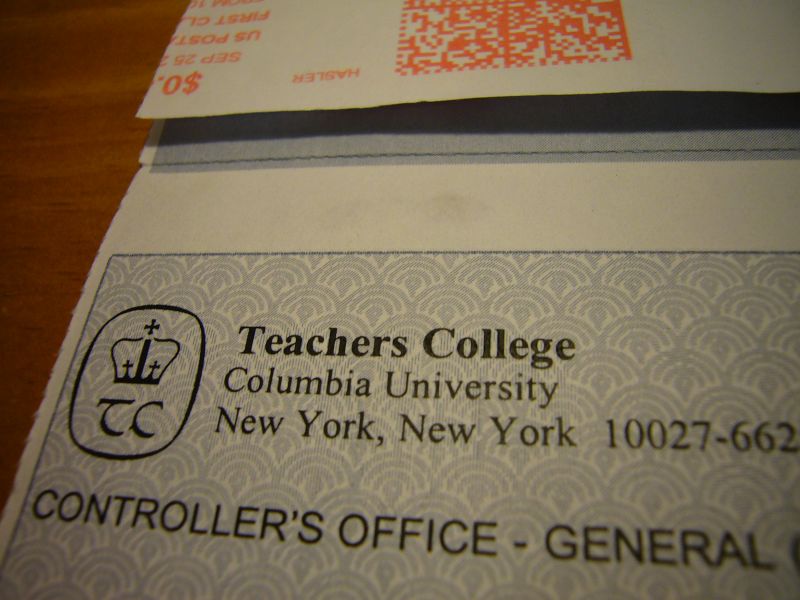This close-up photograph captures the top left corner of a piece of mail, likely a letter or check from Teachers College, Columbia University in New York, NY 10027-662. The mail rests on a wooden table and features a blue and white patterned background with repeated arc shapes. Prominently displayed is a logo: a crown with three crosses and the initials "TC" enclosed in an oval shape, next to the text "Teachers College, Columbia University, New York, New York." Beneath this is printed "Controller's Office General." An orange barcode is visible at the top of the image, signifying postage information. Some details are cut off due to the close-up nature of the photograph.